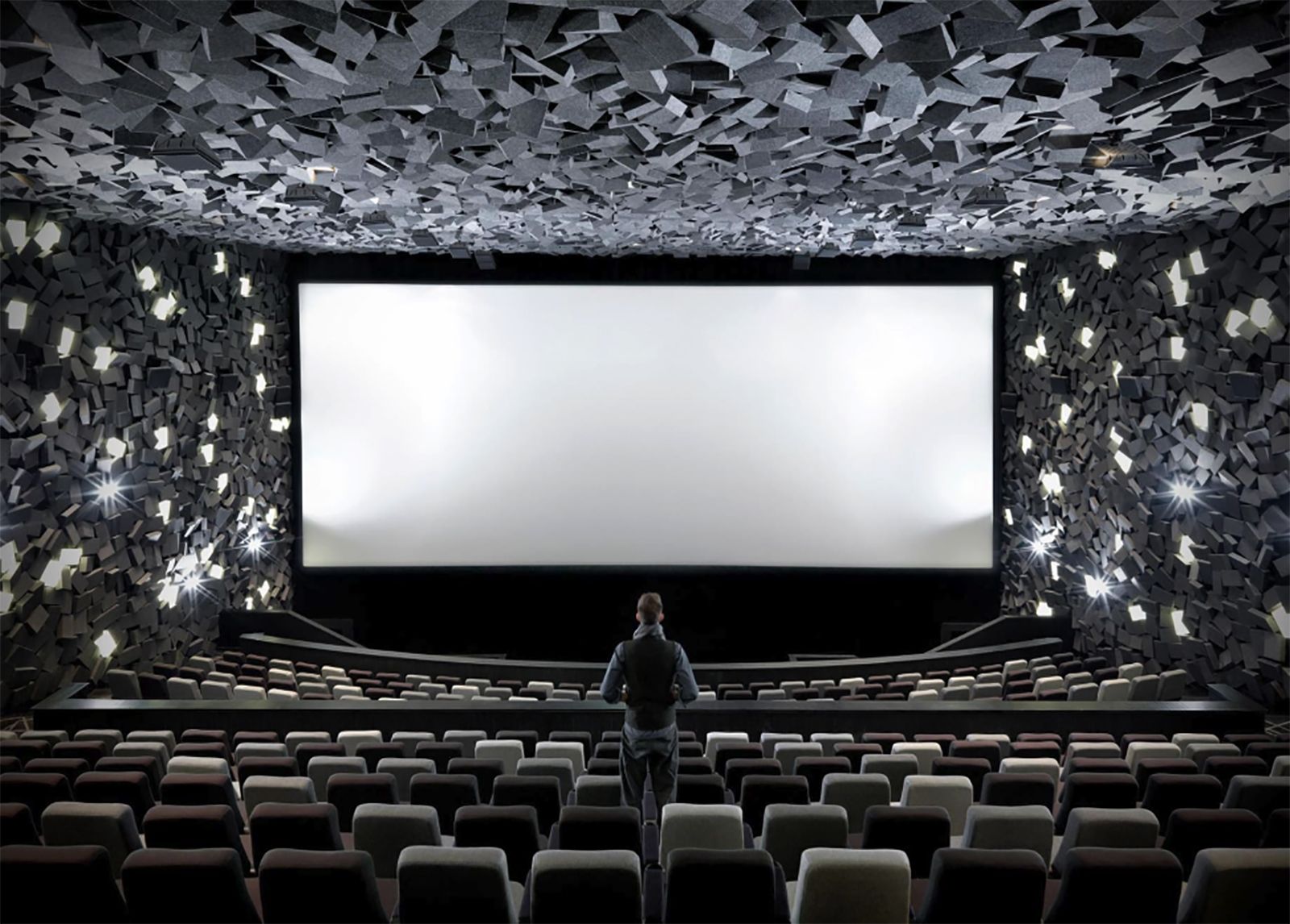This is a detailed, computer-generated 3D render of the interior of a large movie theater. Dominating the front of the image is a blank, rectangular white screen. The seating area is populated with an assortment of seats in various colors—primarily brown, but also featuring irregular patterns of cream, gray, and black. Positioned in the middle of the seats is a lone man, who appears to have been digitally inserted. He is facing the screen with his back toward the viewer and is dressed in dark attire, including a black vest over a blue dress shirt and blue jeans. 

The theater’s walls and ceiling boast a unique, gravelly texture formed by numerous jagged, irregularly shaped gray structures. Interspersed among these textured surfaces are bright white lights, adding illumination to the left and right walls. The seating sections are divided by short black barriers, further emphasizing the theater’s 3D-rendered nature. Overall, the image showcases the solitude of a single man in a meticulously detailed and uniquely designed digital theater environment.